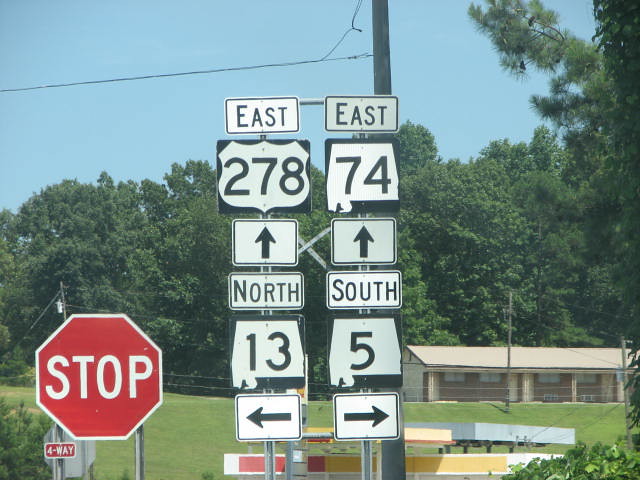The image captures a serene outdoor scene with a light blue sky overhead. Prominently featured are numerous street signs, including a distinctive red stop sign with the word "STOP" written in white, located at the bottom left corner. In the middle of the scene, two rows of street signs extend with a line of five signs on each side. In the background, a lush green field is visible, leading up to a house situated on the back right side of the image. The house is framed by a backdrop of tall, verdant trees, completing the picturesque landscape.